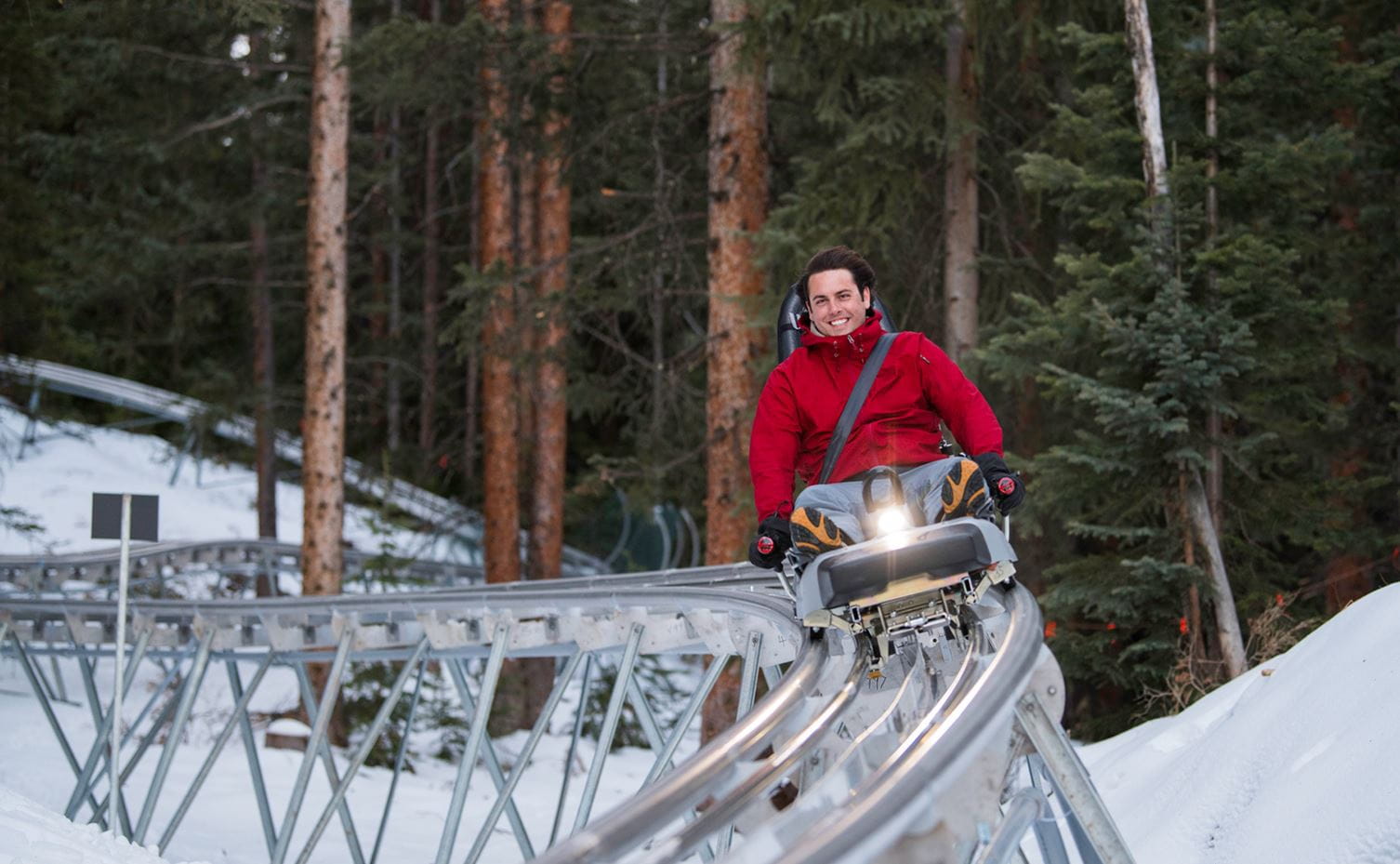The photo captures a man riding a unique, single-rider roller coaster, resembling a sled on a silver, winding track that glides close to the ground and follows the snowy terrain. Surrounded by tall trees blanketed in heavy snow, the man, who has brown hair, is beaming with joy. He wears a thick red jacket, gray pants, and black gloves, gripping the two side handles, likely used as brakes. His seat features a diagonally fastened seatbelt for safety, and a frontal light shines directly at the camera. The well-constructed track, made of aluminum, curves and swirls through the picturesque winter landscape, adding to the thrilling adventure.